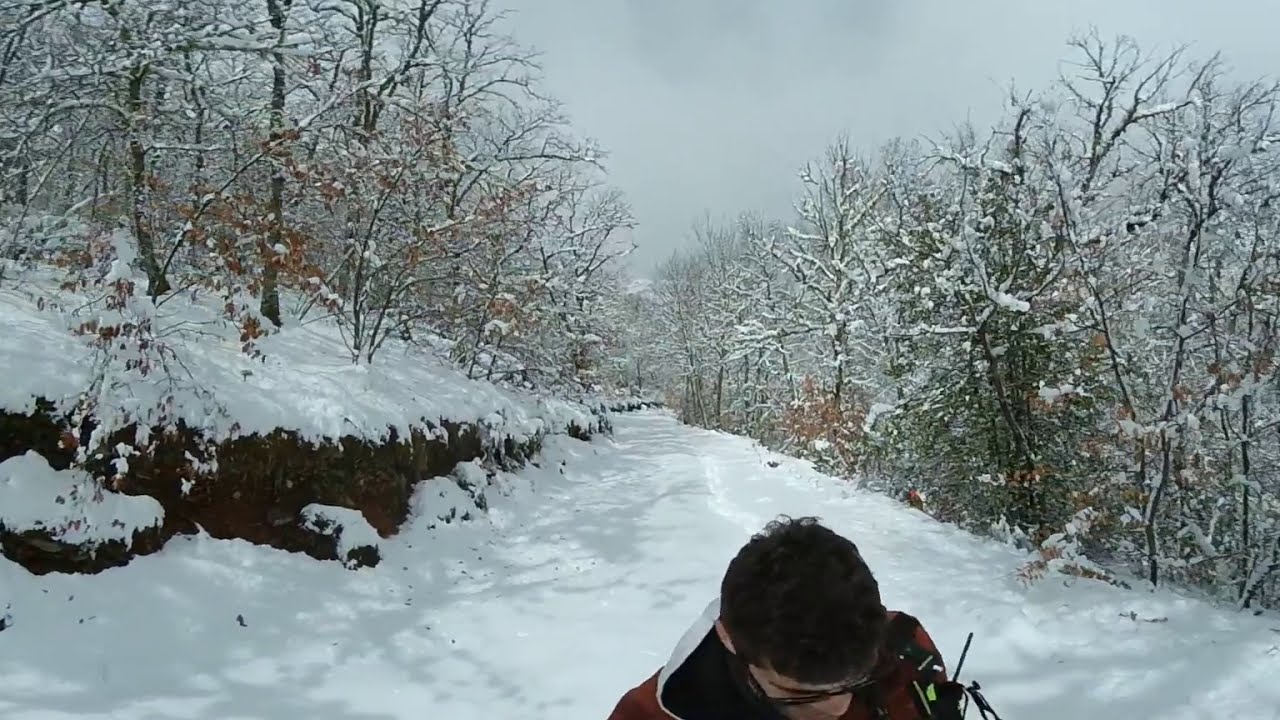In this detailed winter photograph, a man with short dark hair, wearing black glasses and a red coat with a white and black hood, is centrally positioned at the forefront, partially cut off so only the top of his head and shoulders are visible. He appears to be looking down, possibly watching his steps on a snow-covered path. A cord is seen hanging from his coat, suggesting he might be carrying a radio or some other device. 

The background reveals a serene winter landscape. A wide, snow-blanketed trail extends behind him, marked by his footprints. On either side of the pathway, trees are heavily laden with fresh snow, creating a picturesque scene. Most of these trees are barren, devoid of leaves, though some evergreens among them add a touch of green. There are also a few with dead, yellowish-brown leaves, and sporadically some with red leaves and branches.

To the left of the path, a steep hill with exposed brown dirt and rocks rises, contributing to the rugged natural setting. The sky overhead is a dull gray, reflecting the cold, overcast ambiance of a wintry day. The entire setting conveys a cold, tranquil atmosphere typical of a snowy woodland scene.